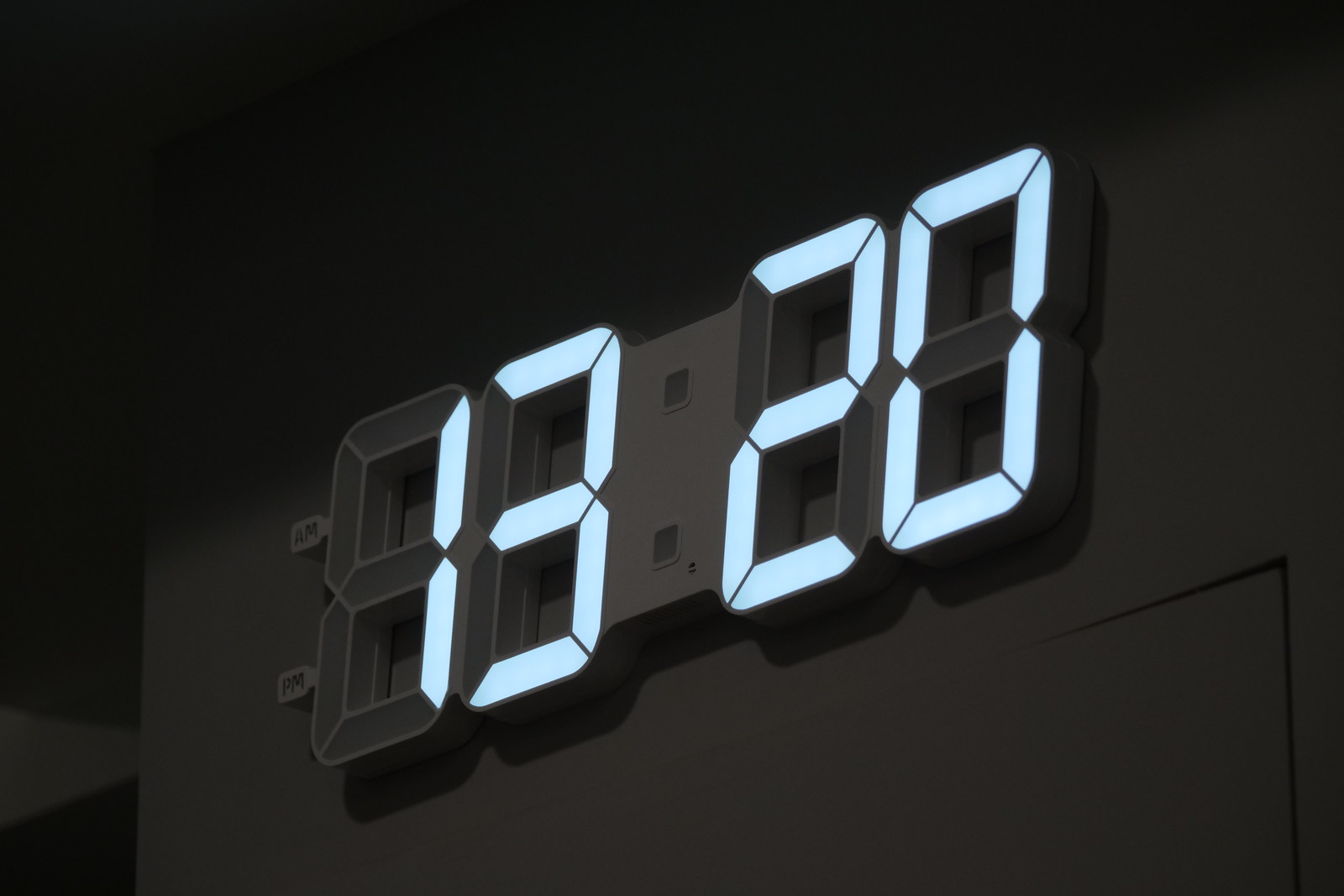This photograph features a digital clock prominently mounted on a wall, displaying the time in military format as 1320 hours (1:20 PM). The clock's sleek white design contrasts with the dim lighting of the environment, which is particularly noticeable in the upper left corner of the image where the shadowing creates a darkened effect. The clock's display is divided by a central space housing two vertically aligned squares, with two digits on each side of this space. The left side of the display contains a sticker divided into two sections, with "AM" on the top half and "PM" on the bottom half, adjacent to the hour digits. The clock is positioned above a doorway, evidenced by a visible door frame and crevice just beneath the clock.